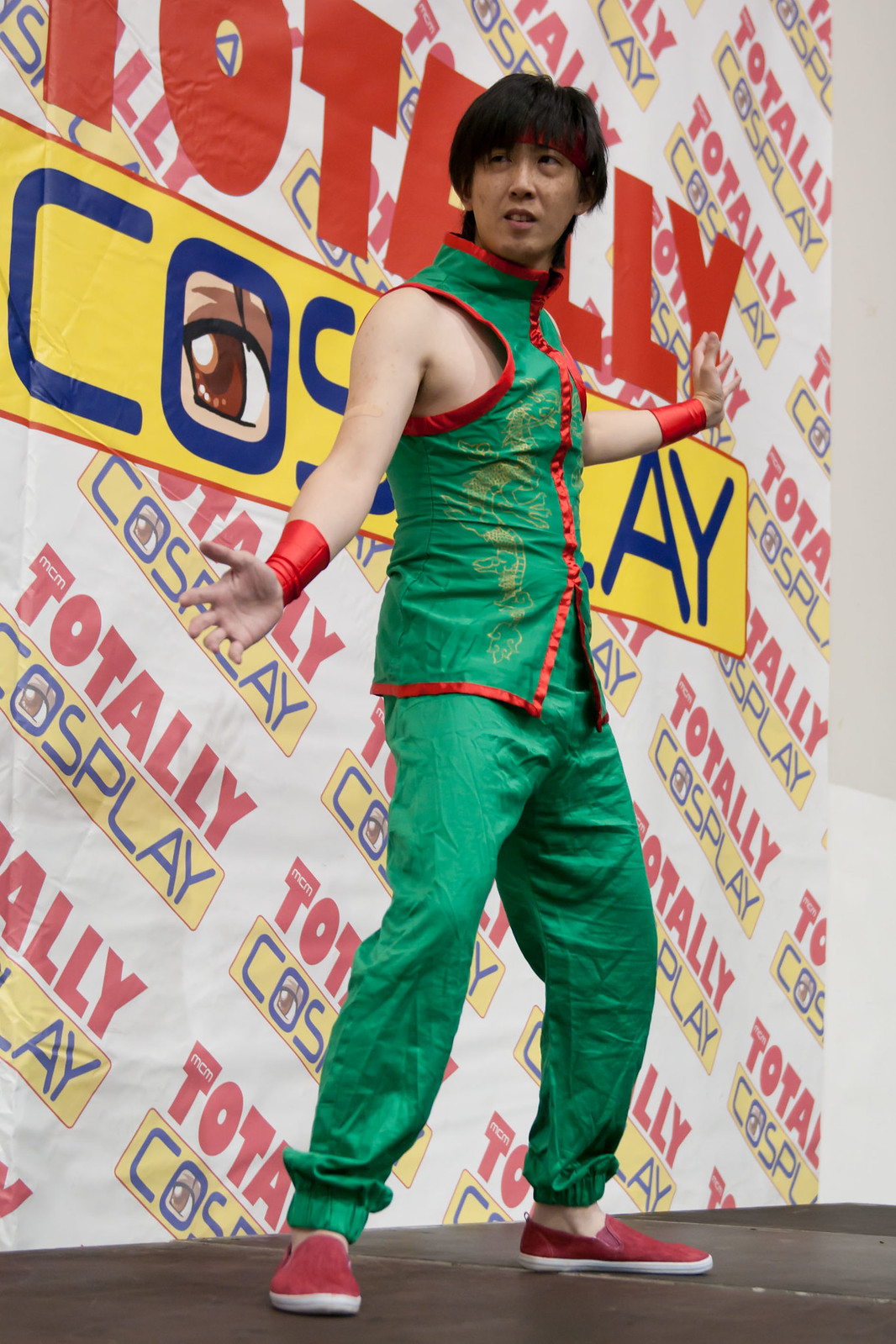In this indoor photo, presumably at a cosplay convention, we find an Asian man dressed in a green outfit with red trim, red armbands, and red shoes, complemented by a red bandana on his forehead. His dark hair is styled in a bowl cut. The shirt features gold designs that might depict a tiger or a dragon, though it's not entirely clear from the angle. The stage he's standing on is hard and platform-like. Behind him, the backdrop displays the words "Totally Cosplay" in various formats and sizes. "Totally" is written in red, and "Cosplay" appears in blue over a yellow banner, with the "O" creatively depicted as a stylized anime eye. The setting suggests a lively atmosphere typical of a cosplay event.